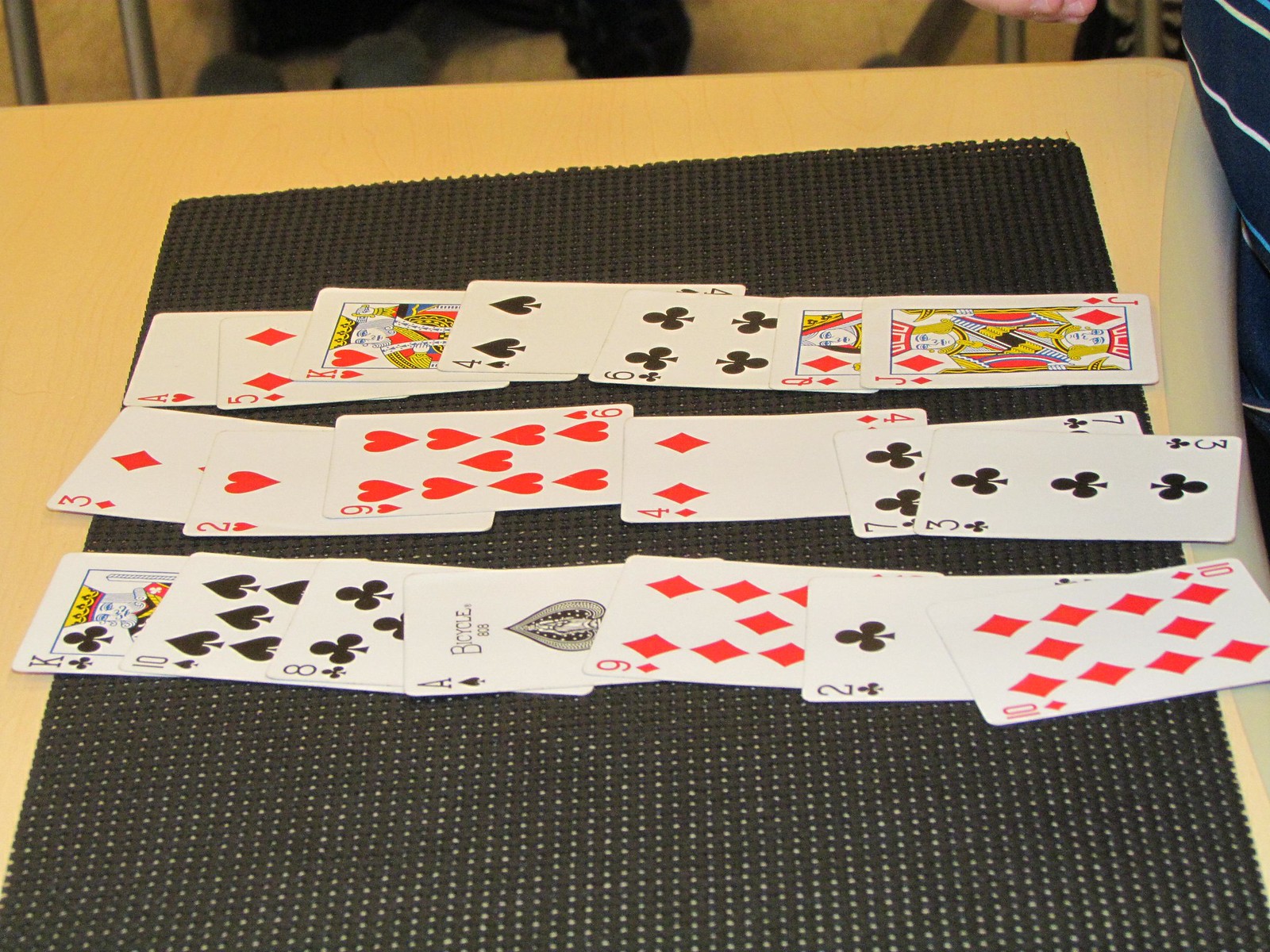In this color photograph, a table or counter of a yellowish-white hue is adorned with a brown mat featuring numerous tiny white dots. Arranged in three horizontal rows, playing cards are meticulously displayed across the mat. In the top row, extending horizontally from left to right, are the Ace of Diamonds, Five of Diamonds, King of Hearts, Four of Spades, Six of Clubs, Queen of Diamonds, and Jack of Diamonds. The middle row showcases the Three of Diamonds, Two of Hearts, Nine of Hearts, Four of Diamonds, and Seven of Clubs. The bottom row presents the King of Clubs, Ten of Spades, Ace of Spades, Nine of Diamonds, Two of Clubs, and Ten of Diamonds. No players are visible; the cards appear to have been temporarily abandoned. At the very top of the image, beyond the table, a couple of gray bars are visible on the left side, alongside a black object. On the right edge, a small sliver of a pink object is also visible.